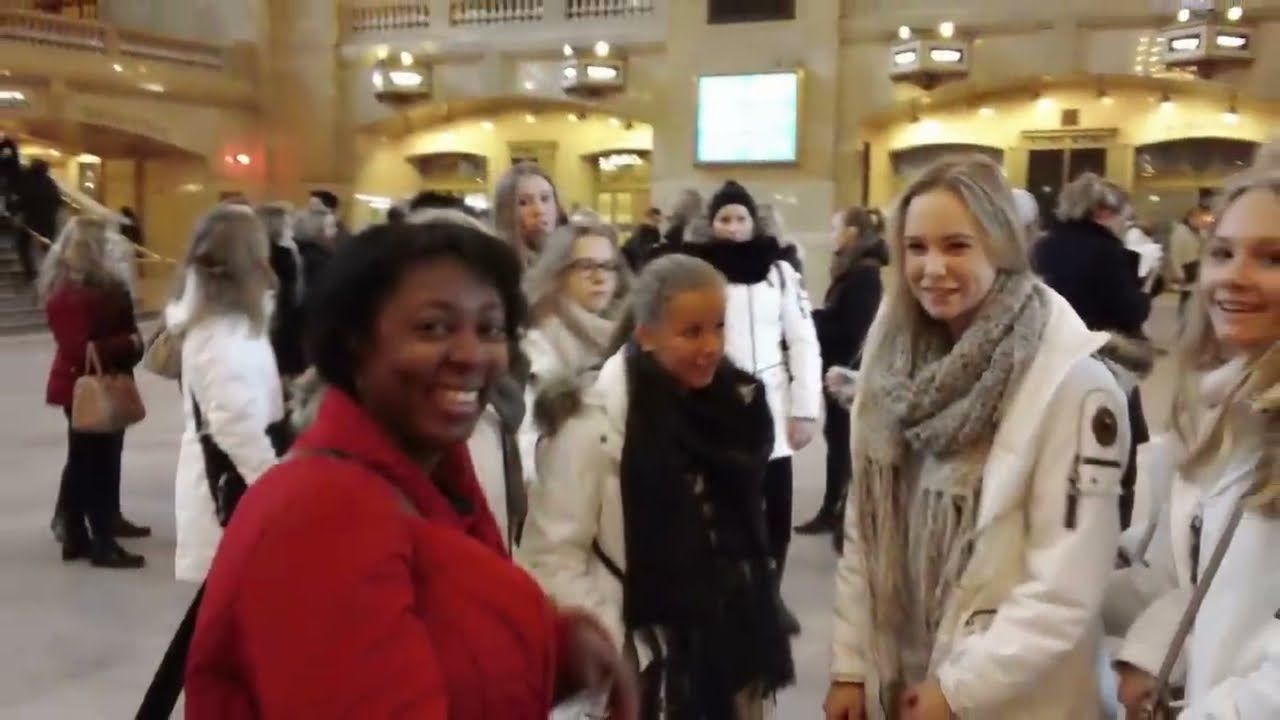In a blurry, low-resolution image that seems captured in motion, possibly from a video, we see a bustling scene, likely in an upscale, grand location such as Grand Central Station or a large hotel lobby. The central focus is a group of four women standing amidst a larger crowd, predominantly female, many of whom are dressed similarly in winter outfits. 

The scene features mostly women wearing thick white jackets paired with either light gray or black scarves. The central figure closest to the camera is notably distinct: an African-American woman wearing a bright red jacket, her short black hair framing a smile that reveals her top teeth. She has a black strap slung over her shoulder, and her left hand is raised and bent towards the ground.

To her immediate right stands another woman, the only one among the close four not looking at the camera. She is shorter, with grayish hair and is dressed in a white coat with a black scarf reaching her waist. Next to her is the tallest woman, a white woman with dirty blonde hair, a grayish scarf, and a black circular logo with a dangling strap on her left shoulder. The fourth woman, who partially faces the camera, has part of her face cut off on the right side of the image. She, too, is wearing a white coat with a handbag strap crossing from her right shoulder downwards.

The backdrop includes elements like arches, doors, screens, walls, and possibly stairs, adding to the sense of a spacious, upscale environment. Despite the blur and low light, the image captures vivid colors including red, white, black, tan, and gold, reinforcing the wintery, coordinated appearance of this intriguing gathering.